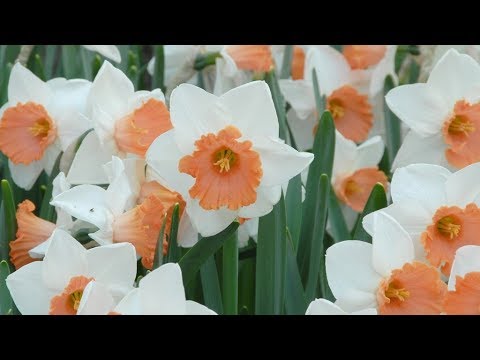This rectangular photograph, bordered by black at the top and bottom, captures a close-up of approximately a dozen trumpet-shaped flowers, each with long green stems and oblong, flat, dark green leaves. The flowers exhibit distinctive white petals that transition into vibrant orange and peach hues towards their centers, evocative of a trumpet vine or bulb-like plant. The central area of each bloom features yellow, possibly pollen, adding a contrasting focal point against the orange segments. The image, likely taken during daylight, sharply focuses on these flowers, emphasizing their unique coloration and structure while excluding any other background elements.